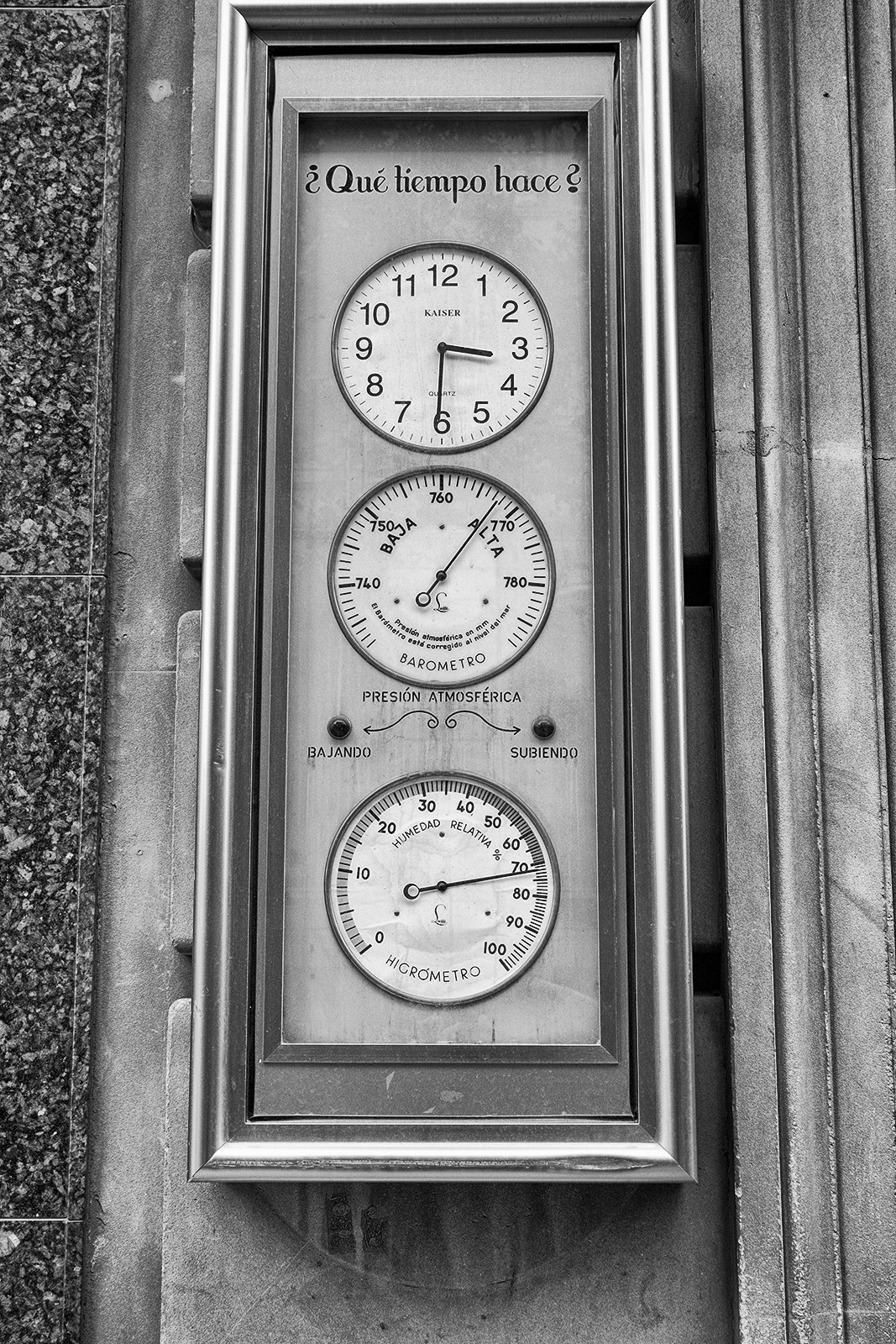A black and white photograph captures a rectangular frame that houses three equally sized circular analog displays. The leftmost circle features a classic clock with hour, minute, and second hands. The center circle is a barometer, designed to measure atmospheric pressure with a similar needle mechanism. The rightmost circle is a hygrometer, indicating humidity levels with meticulous precision. Each gauge is intricately detailed, showcasing the fine craftsmanship of these analog instruments.